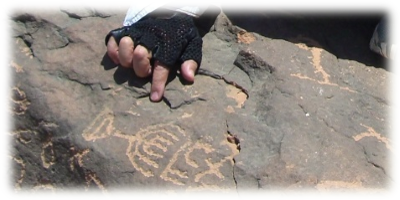The image is a small, rectangular photograph taken outdoors in the daytime and seems to have been slightly digitally altered. At the center of the composition is a large, grey and brown rock featuring intricate carvings and engravings. Prominent among these engravings is a detailed depiction of a menorah, positioned toward the middle-left of the rock. Additional carvings include various letters and a large, yellow pattern resembling a sideways cup with an X-mark, located at the bottom center of the image.

A person's hand, clad in a black glove with the fingertips exposed, is seen pointing directly at the menorah. The hand appears at the top-left middle section of the photograph. The blurred edges of the photograph and the meticulous carvings on the rock suggest that this might be a significant archaeological find, sparking interest and curiosity in the person pointing.